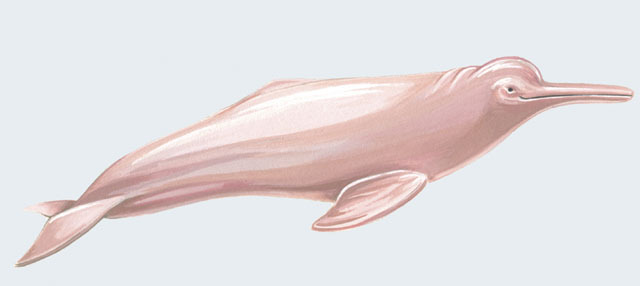The image is an illustration of a unique sea creature resembling an Amazon pink dolphin, though the colors and artistic style deviate from a realistic portrayal. The creature's body features a shiny, nearly nude tone that appears dull with a subtle sheen, with shades shifting into hints of pink and mauve. This artistic rendering showcases a classic elongated beak-like mouth, devoid of visible teeth, with a certain platypus-like quality. From the side, we see its small, black pupil set in a sweet-looking eye, and a slightly bulbous forehead. The creature’s back has a slight hump highlighted in white, and it possesses stubby fins on the side and a tail at the back, enhancing its dolphin-like silhouette. The background is a pale lilac-gray, providing a soft contrast to the creature’s muted yet captivating coloration.